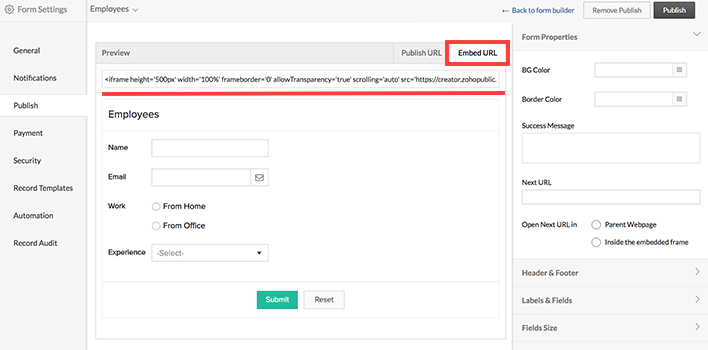This screenshot showcases a computer application with a meticulously structured layout. On the left, a light gray sidebar features various settings options. At the top left, a medium gray cog icon signifies settings, followed by "Form Settings" in medium gray text. Directly below, a thin medium gray horizontal line separates this section from a list of dark gray text options, such as General, Notifications, Publish (which is highlighted in a white rectangle with light gray horizontal lines at the top and bottom), Payment, Security, Record Templates, Automation, Record, and Audit.

The highlighted Publish option connects to the main body of the page on the right, which has a white background. At the top of this main section, a light gray header spans the width of the page. To the left within this header, next to "Form Settings," the word "Employees" appears in dark gray, accompanied by a dark gray arrow pointing downwards. Toward the far right of this header, blue text reads "Back to Form Builder," flanked by a blue left-pointing arrow. Further right, a light gray box outlined in dark gray contains the text "Remove Publish" in dark gray. Adjacent to this box, a dark gray rectangle with rounded corners displays the word "Publish" in white text.

In the main content area, another light gray header indicates the section's title. On the left side, "Preview" is written in dark gray text, followed by a significant amount of negative space. A vertical medium gray line divides this space from "Publish URL" in dark gray text toward the far right. Below this, "Embed URL" is written in black text on a white background, highlighted with a surrounding red box.